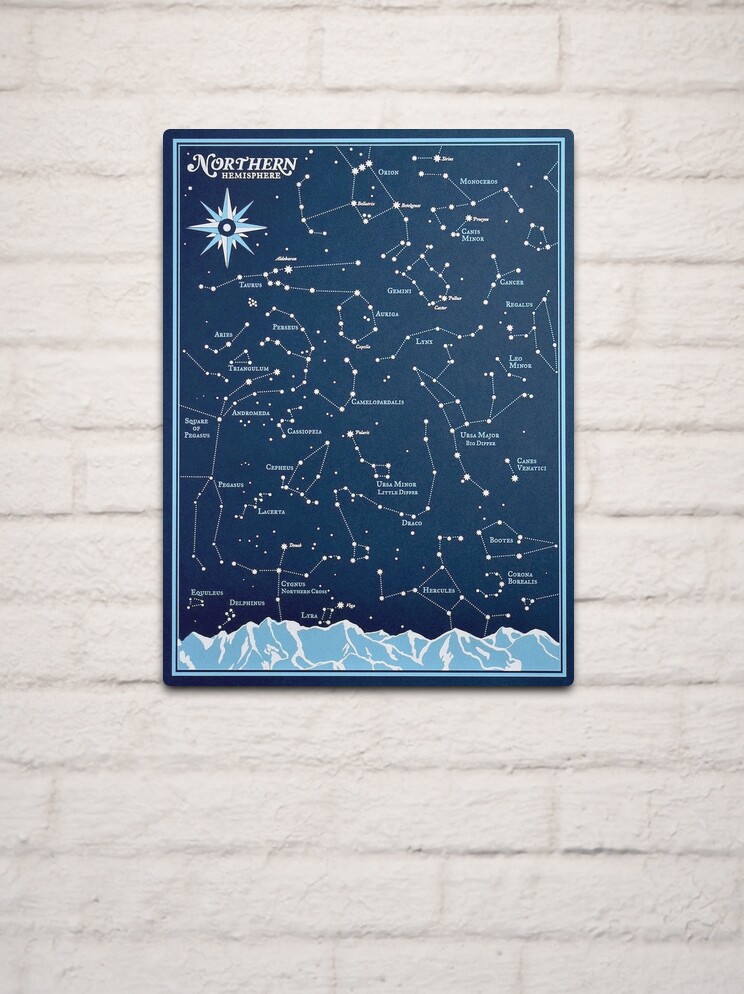The image depicts a poster mounted on a white-painted brick wall. The poster features a dark blue night sky framed by two lighter blue bands. At its base, there is a silhouette of mountains in shades of white and light blue. The top left corner of the poster is labeled "Northern Hemisphere," accompanied by a stylized compass logo in blue and white. The majority of the poster showcases various constellations and star formations visible in the Northern Hemisphere, with each constellation's stars interconnected by lines and labeled with their respective names. There appear to be around a hundred stars or points forming these patterns, meticulously plotted to represent their actual positions in the night sky.